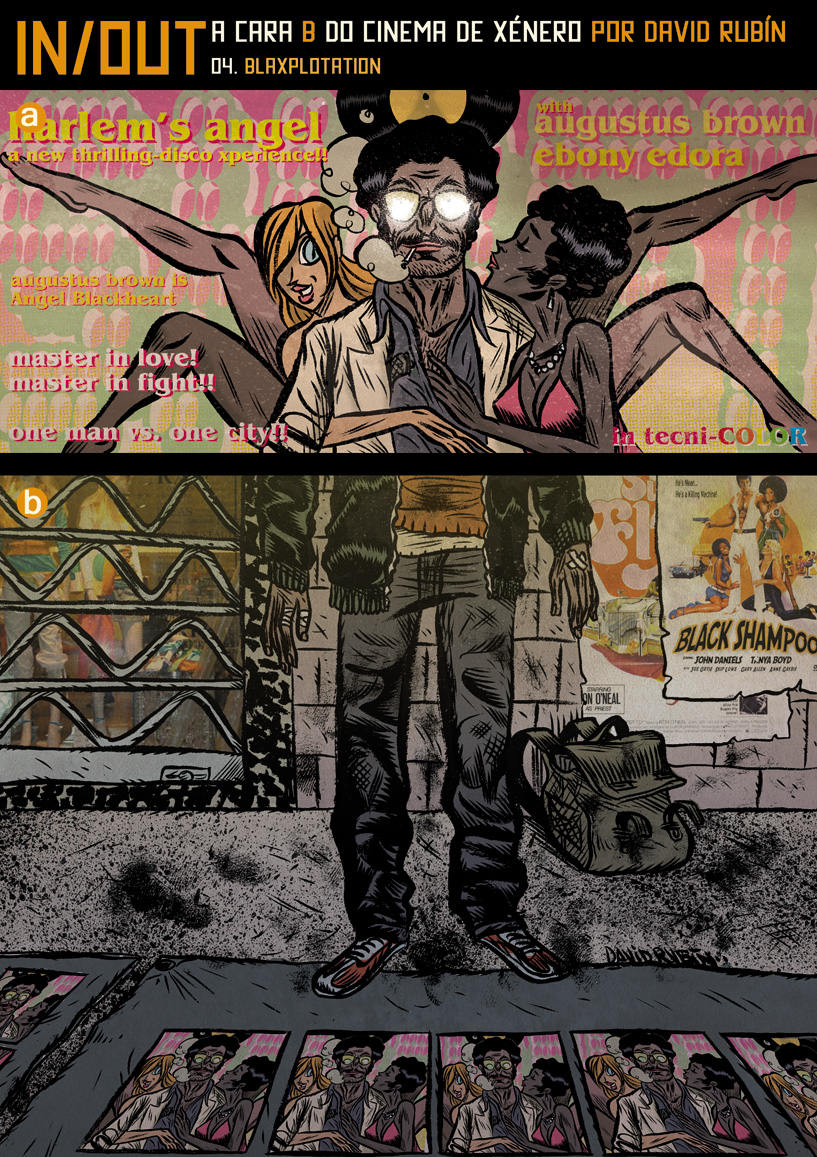This animated poster features a visually striking, cartoonish depiction reminiscent of comic book art. Dominating the top in bold, orange slashed-out text, it reads: "In/Out Akara BDD Cinema de Zanero for David Rubin." Below this, in vibrant yellow letters, the title "Harlem's Angel" and further text promote "Augustus Brown and Ebony Adora," hinting at a thrilling disco adventure. The central figure is a stylish black man wearing white sunglasses, exhaling smoke from a cigarette. To his left stands a red-haired woman, and to his right, an African American woman wearing a red bra kisses him. The upper left corner proclaims, "Harlem's Angel: A new thrilling disco experience," suggesting a lively and dramatic narrative.

Additional tagline text states: "Master in love, master in fight. One man versus one city. High technical," implying complexity in both romantic and combative themes. Behind the main characters, there's a vinyl record present, hinting at a musical element. The bottom half of the poster, cast in darker hues, reveals the man’s worn jeans, old red shoes, and a backpack on the ground beside him.

To the right, a translucent poster with the title "Black Shampoo" and additional character illustrations is displayed over a wall drawing. There is also a depiction of the same man on a sidewalk with a blanket covered in posters, evoking a gritty, urban ambiance.